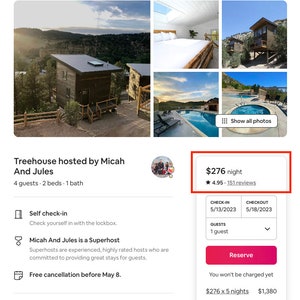**Detailed Caption:**

This image is a screenshot captured from a mobile phone display. At the top of the screen is a collection of pictures. There is a large photograph positioned on the left, accompanied by four smaller images arranged in a grid on the right. Below these images, the text reads "Treehouse hosted by Micah and Jules." Additional details indicate that the accommodation can host four guests and includes two beds and one bath. On the right side of this text, there is a profile picture. Further to the right, the text indicates a rate of $276 per night, and it shows a rating of 4.95 stars based on 151 reviews. 

Additionally, a digitally added red rectangle outlines the information that displays the nightly rate and reviews. At the bottom of the image, it states that the property offers self-check-in, highlights Micah and Jules as super hosts, and mentions that there is free cancellation available before May 8th. To the right side of this section, there is a small boxed area detailing the check-in and check-out dates, the number of guests, and also includes a prominent red "Reserve" button for booking the stay.